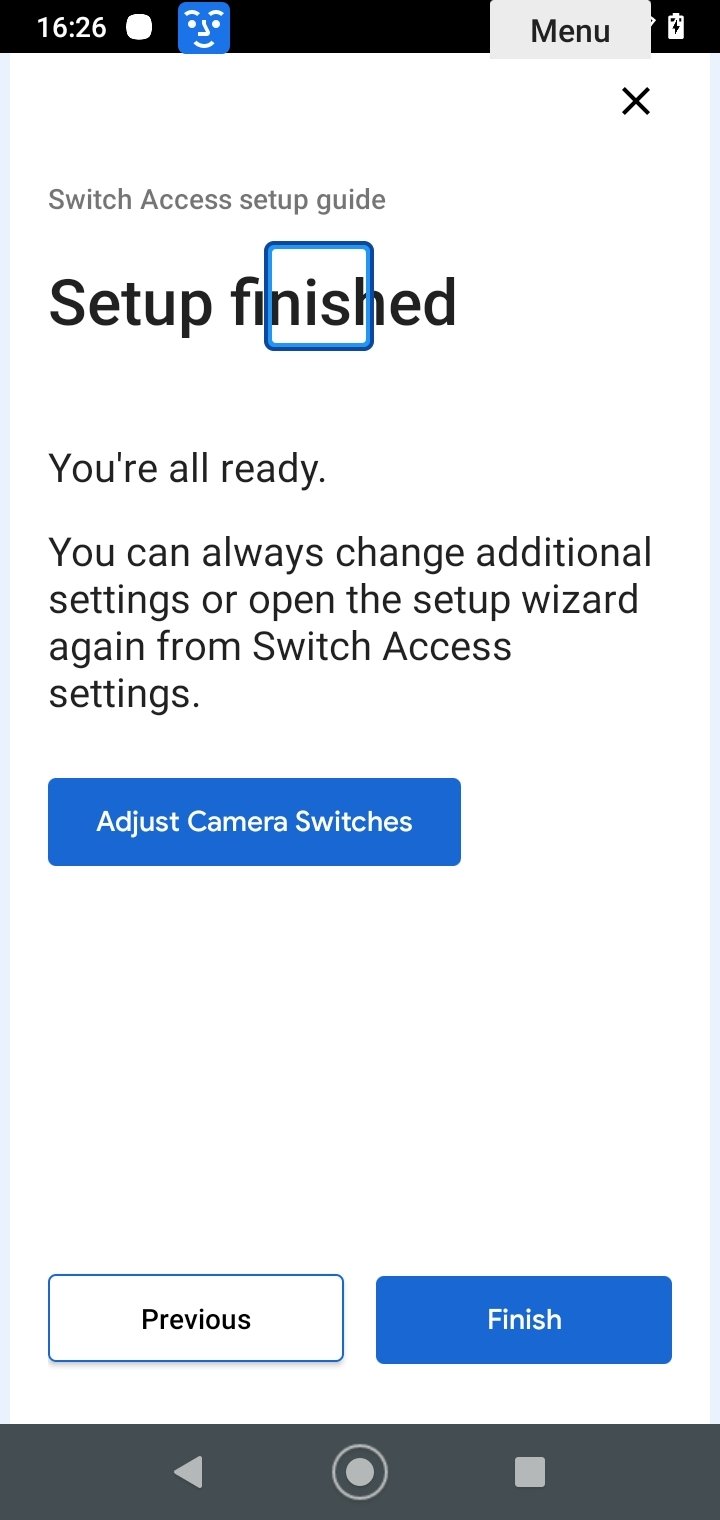This is an image captured from a cell phone screen showing a "Switch Access Setup Guide" at 16:26. The interface features a predominantly white-themed layout. At the top, there's a white box displaying the menu options. Below it, a notification area includes a white message indicator. The central part of the screen prominently reads "Switch Access Setup Guide" with a subheading, "Setup Finished," highlighted within a blue box, and the text "You're all ready. You can always change additional settings or open the setup wizard again with switch access settings" beneath it.

Midway through the screen, there's another blue box labeled "Adjust Camera Switches." Further down, towards the bottom, the phone has navigation options with "Previous" in a white box outlined in blue, and "Finish" in a blue box, indicating navigation through the setup process.

At the very bottom of the screen, within a black navigation bar, there are three light gray icons: a left-pointing arrow on the left, a circled icon in the center, and a square on the right. These icons are outlined in white, helping to distinguish them from the black background of the navigation bar. This detailed description completes the overview of the cell phone screen's displayed setup page.